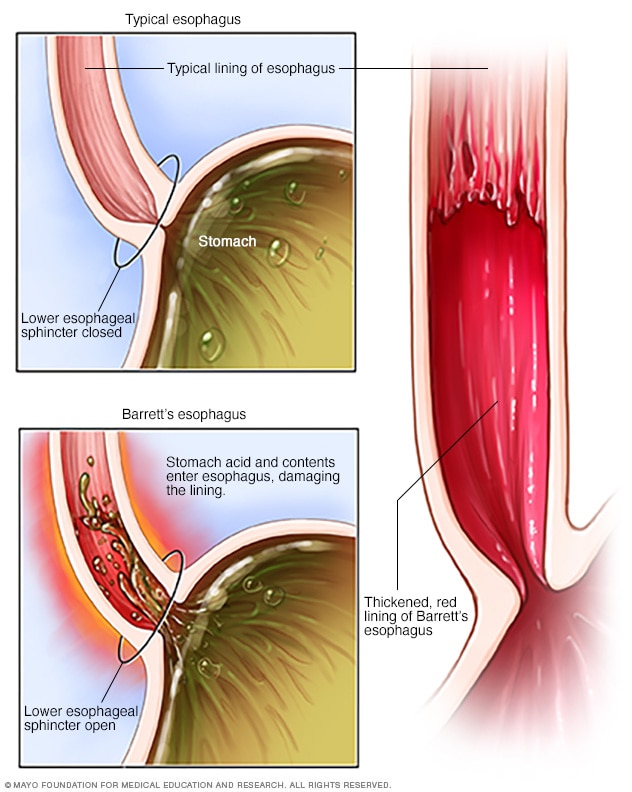This copyrighted medical illustration from the Mayo Foundation for Medical Education and Research provides a detailed comparison between a typical esophagus and one affected by Barrett's Esophagus. The upper section of the image depicts a normal esophagus with its characteristic pink lining, a closed lower esophageal sphincter, and the stomach positioned below it. This closure of the sphincter effectively prevents stomach acids and contents from entering the esophagus. In contrast, the lower section showcases Barrett's Esophagus, where the lower esophageal sphincter remains open, allowing stomach acids and contents to flow back into the esophagus, damaging the lining. This damage is illustrated by the thickened and red lining characteristic of Barrett's Esophagus. Additionally, text annotations within the diagrams explain the mechanism and detrimental effects of acid reflux, highlighting the distinction between the healthy esophageal structure and the pathological changes seen in Barrett's Esophagus.